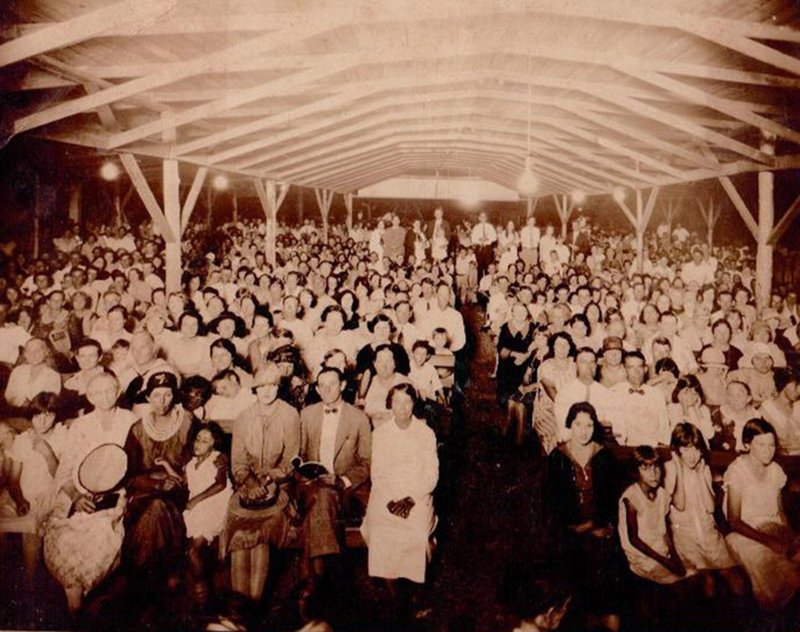The black-and-white photograph, likely dating from the 1930s to early 1950s, captures a densely packed, outdoor pavilion event held at night. Illuminated by bare light bulbs hanging from wires, the scene reveals hundreds of people seated in pew-like arrangements, facing the camera. Their attire, reminiscent of Sunday best, suggests a formal occasion, possibly a revival meeting or religious service. The wooden structure overhead lacks walls, akin to a covered picnic area. The crowd is diverse, with children and adults predominantly sporting dark hair, contributing to the historic ambiance captured in this faded, Polaroid-style image.